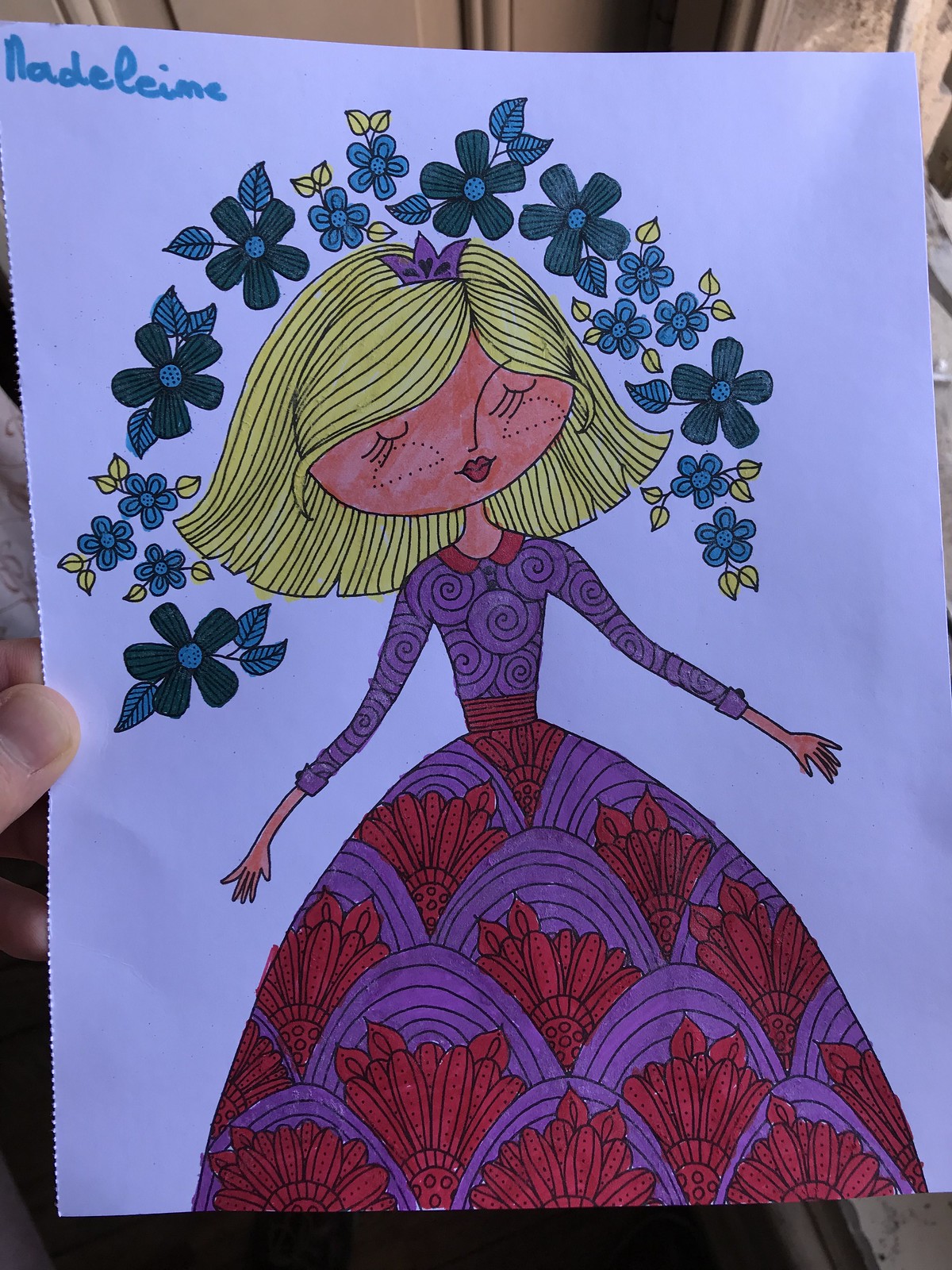In this captivating illustration, set against a pristine white sheet of paper, vibrant hues of pink, purple, red, blue, green, and yellow come to life. A hand, with the thumb and index finger visible, holds up the paper, drawing attention to the beautifully detailed artwork. 

In the upper left-hand corner, the name "Madeline" is inscribed, introducing us to the central figure of the drawing: a girl with flowing, shoulder-length blonde hair. She is dressed in an intricately designed purple dress that extends to her wrists and billows outwards from the waist in a graceful, poofy silhouette.

The top of the dress features a sophisticated pattern of black swirls against a purple backdrop, seamlessly transitioning into a rainbow-inspired design at the bottom, though dominated by shades of purple. Adding to the dress's charm are delicate red floral patterns that adorn the fabric.

Surrounding Madeline's head is a whimsical border of flowers, interwoven with green and teal petals and yellow-leaf accents, enhancing the enchanting aura of the drawing. This detail-rich artwork reflects both creativity and a keen eye for artistic expression.